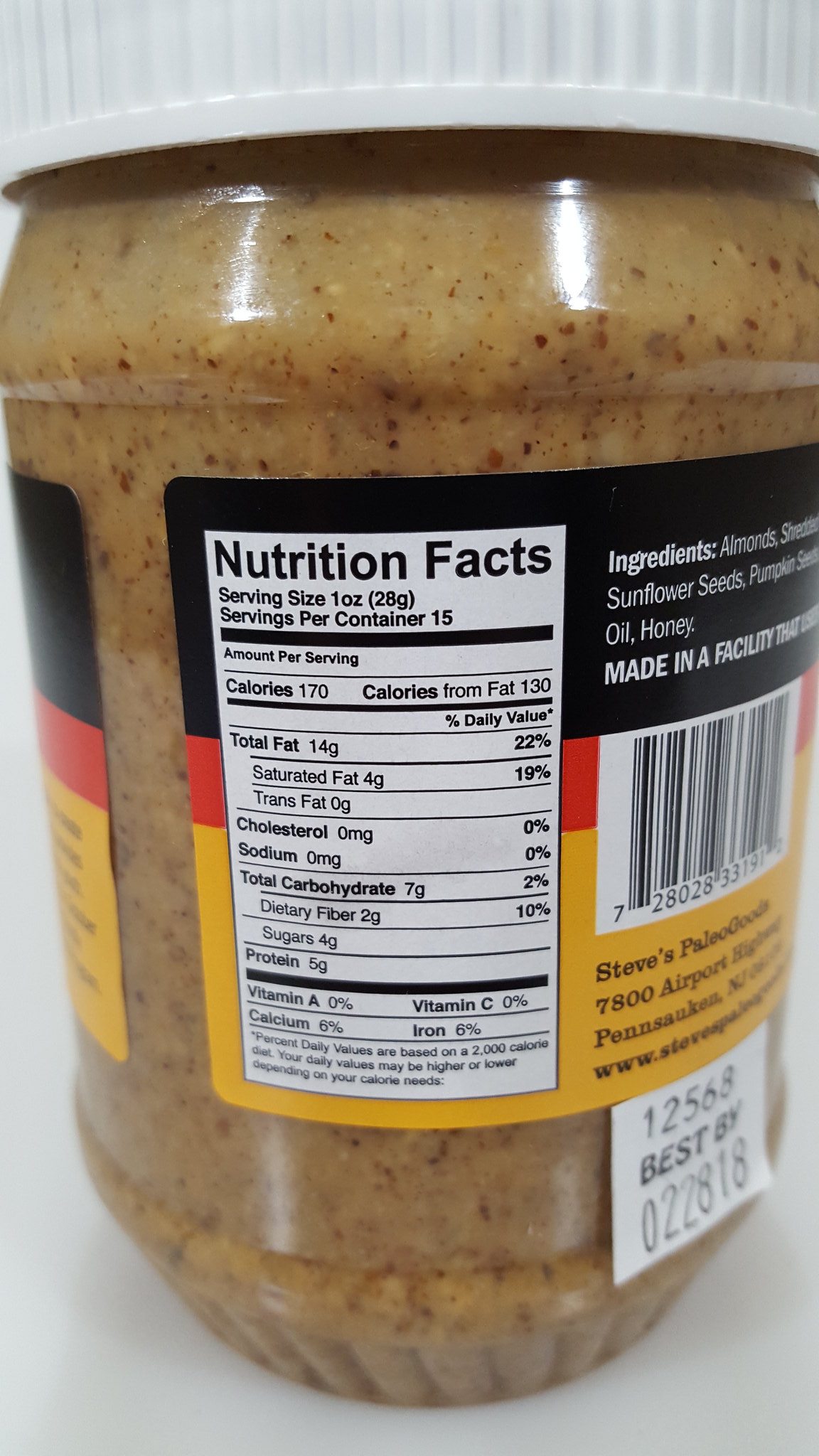The image features a close-up of a clear plastic jar with a white screw-on lid, containing a brownish substance with specks of darker brown inside, identified as almond butter. Prominently displayed on the side is a detailed label in black with red and yellow stripes, highlighting the nutrition facts. The label indicates that the almond butter contains 170 calories per serving with 15 servings per container. The nutritional breakdown includes 14 grams of total fat, 0mg of cholesterol and sodium, 7 grams of total carbohydrates, and 5 grams of protein per serving. Other visible details on the label are the ingredients—almonds, sunflower seeds, pumpkin seeds, oil, and honey—a barcode, the company name "Steve's Paleo Goods," and a sticker displaying the best buy date.